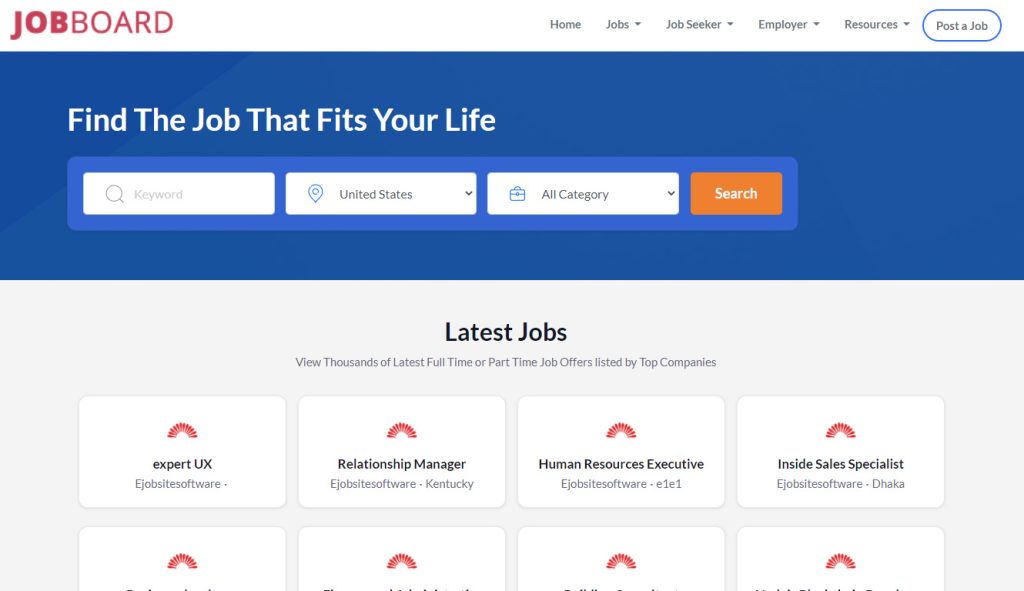This image is a detailed screenshot of a job board website, showcasing various elements. In the top left corner, the word "job board" is displayed, with "job" in bold and both words in red. To the right of this, a horizontal menu is present, featuring the options: "Home," "Jobs" (with a dropdown button), "Job Seeker" (with a dropdown button), "Employer" (with a dropdown button), and "Resources" (with a dropdown button). Additionally, there is a button labeled "Post a Job," encircled by a thin blue line.

Beneath the menu, a large blue box captures attention with the title "Find the job that fits your life" in white text. This blue box also contains a search bar for keyword entry. Adjacent to it, there's a dropdown menu for selecting a location, with "United States" currently chosen, followed by another dropdown menu labeled "All Category." A prominent orange button labeled "Search" is positioned to facilitate the job search.

Below this, a grey background area titled "Latest Jobs" in bold black lettering provides further information, stating "Thousands of latest full-time or part-time job offers listed by top companies." Within this section, eight clickable boxes are displayed, although only the top four are fully visible. These boxes, each featuring a red rainbow-like symbol, detail various job listings:
1. Expert UX | e-jobs | e-jobsite software
2. Relationship Manager | e-jobsite software | Kentucky
3. Human Resources Executive | e-jobsite software | E1E1
4. Inside Sales Specialist | e-jobs | e-jobsite software | DACA